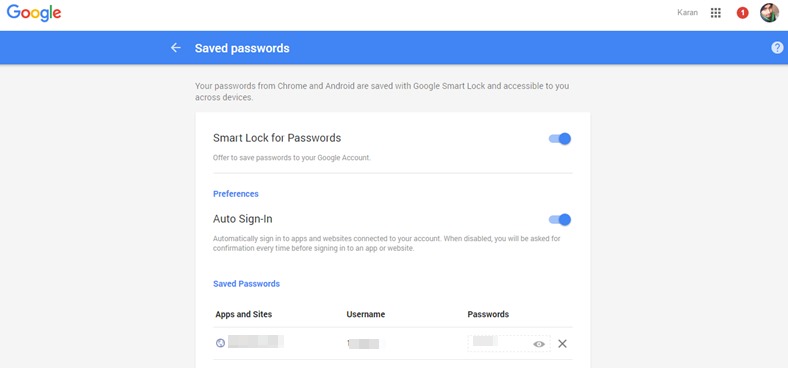This image is a screenshot from a Google interface. At the very top left corner, the recognizable Google logo is displayed, with "Google" spelled out in a distinct combination of colors: a blue "G", red "o", yellow "o", blue "g", green "l", and red "e". 

Towards the top right corner, there is a small profile photo which appears to be of a man who might be of Middle Eastern or Asian descent. Next to the profile photo, a red notification circle with the number "1" is visible, alongside the name "Karan" spelled out in capital letters.

Directly below the header, there is a sky-blue banner. Centered within this banner, a headline reads "Save passwords". Below this headline, a concise explanation states, "Your passwords from Chrome and Android are saved with Google Smart Lock and accessible to you across devices."

The main body of the screen is a white section labeled "Smart Lock for passwords". Underneath this title, the word "Preferences" is shown, followed by the text "Auto sign in", accompanied by an explanatory note in gray font.